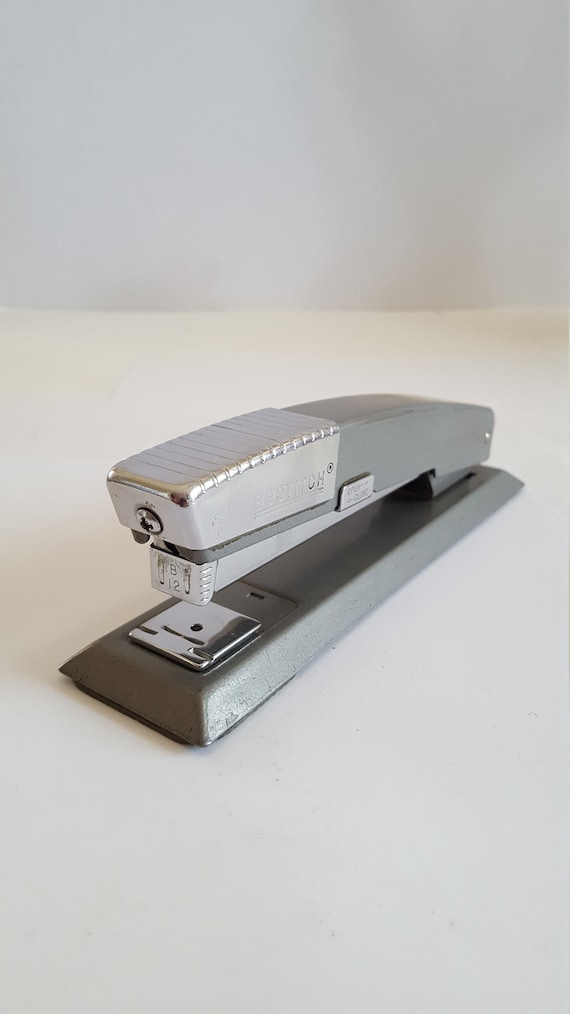This vertically cropped close-up photograph showcases a well-used metal stapler placed centrally on a white surface, possibly a table or tablecloth, set against a white background. The stapler, predominantly gray and silver, is positioned at a diagonal angle facing the bottom left of the image. Its top portion, made of metallic silver, features distinct lines or etching and is fastened with screws. The stapler bears signs of wear, with visible textures and small scratches indicating extensive use. Engraved text, though slightly worn off, can be seen along the top side, alongside the printed letters "B12" on the front part. Light reflections off the metal add to the detailed portrayal of this common, office staple.